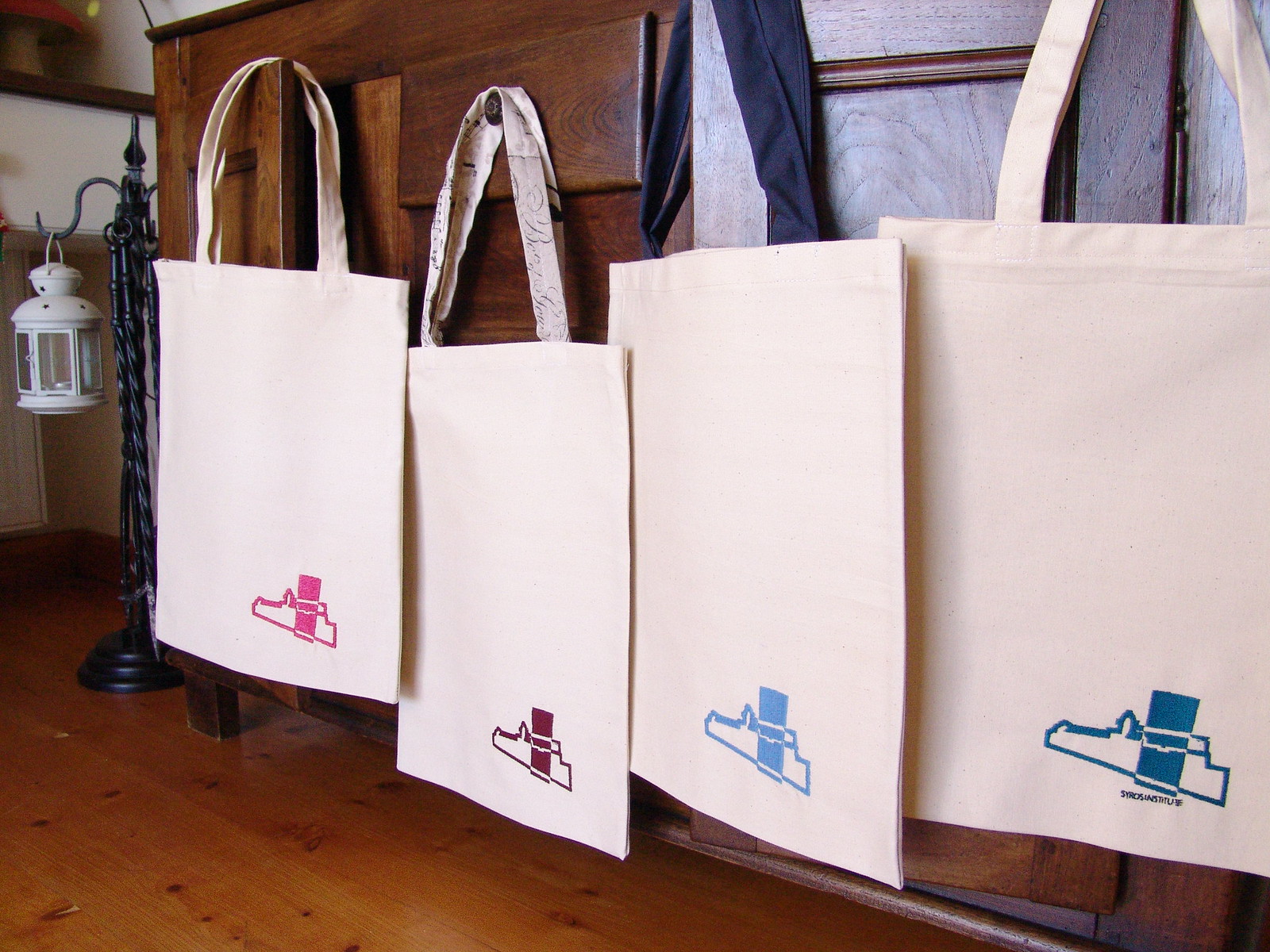In this detailed image inside a house, you see a wooden floor with varying shades of brown and light spots illuminated by light, either natural or artificial. A central dark brown cabinet with slightly open doors and drawers dominates the scene. Four off-white or tan tote bags, each with loop-shaped handles and unique symbols in the bottom right corners, hang on the knobs or doors of the cabinet. The first bag features a pink symbol, the second a brown or maroon symbol, the third a periwinkle blue symbol with black handles, and the fourth a teal or greenish-gray symbol. Underneath each symbol, there is indistinct writing that starts with an 'S'. To the left of the cabinet, a black stand supports a white lantern, contributing to the cozy and eclectic atmosphere of the room.